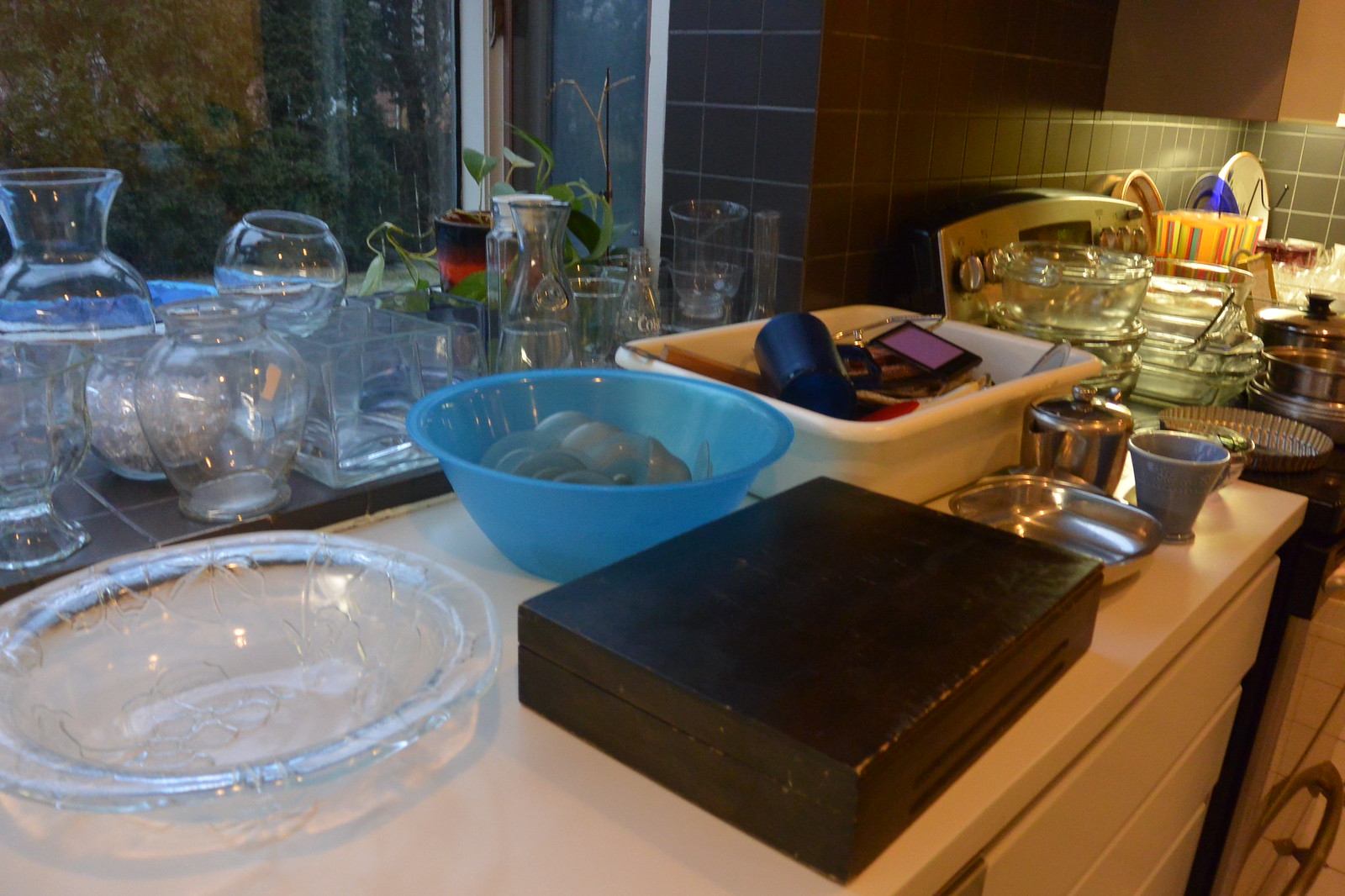In this image, we see a light blonde wood cabinet or countertop featuring several long drawers underneath. The surface of the cabinet is cluttered with various items that suggest a garage sale setting. Among the items, there are multiple glass bowls and flowerpots, including a wide glass ashtray. A blue bowl on the countertop contains some round objects, while a yellow bin is filled with miscellaneous items for sale. Additionally, a solid hardwood box, which resembles an attache case, rests on the surface without any discernible markings. Also visible is a flat, oblong rectangular metal bowl and another blue flowerpot. In the background, there appears to be a bookcase stacked with books or possibly record albums, further indicating the scene is likely a garage sale with a variety of items on display.